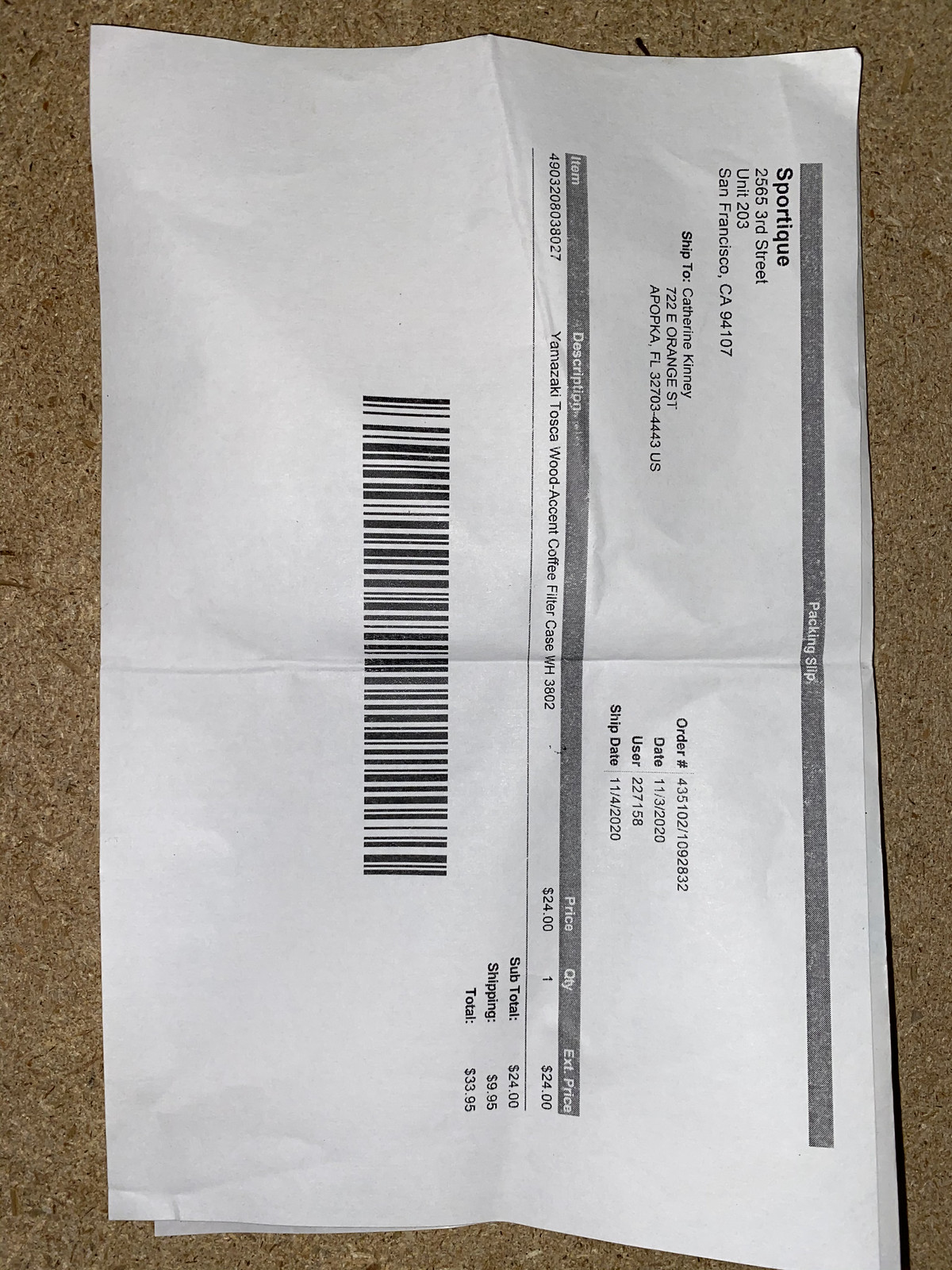The photograph captures a slightly wrinkled and folded invoice from Sportique, a company based in San Francisco. The document, printed on white paper with black ink, details a product delivery, including a ship-to address, an order number, the date, and the ship date. Listed within the contents are the name of the item and the total cost with shipping. At the bottom, a black and white barcode is clearly visible. The invoice is creased both horizontally and vertically, indicating it has been folded and reopened multiple times. The paper lies on a textured corkboard surface.